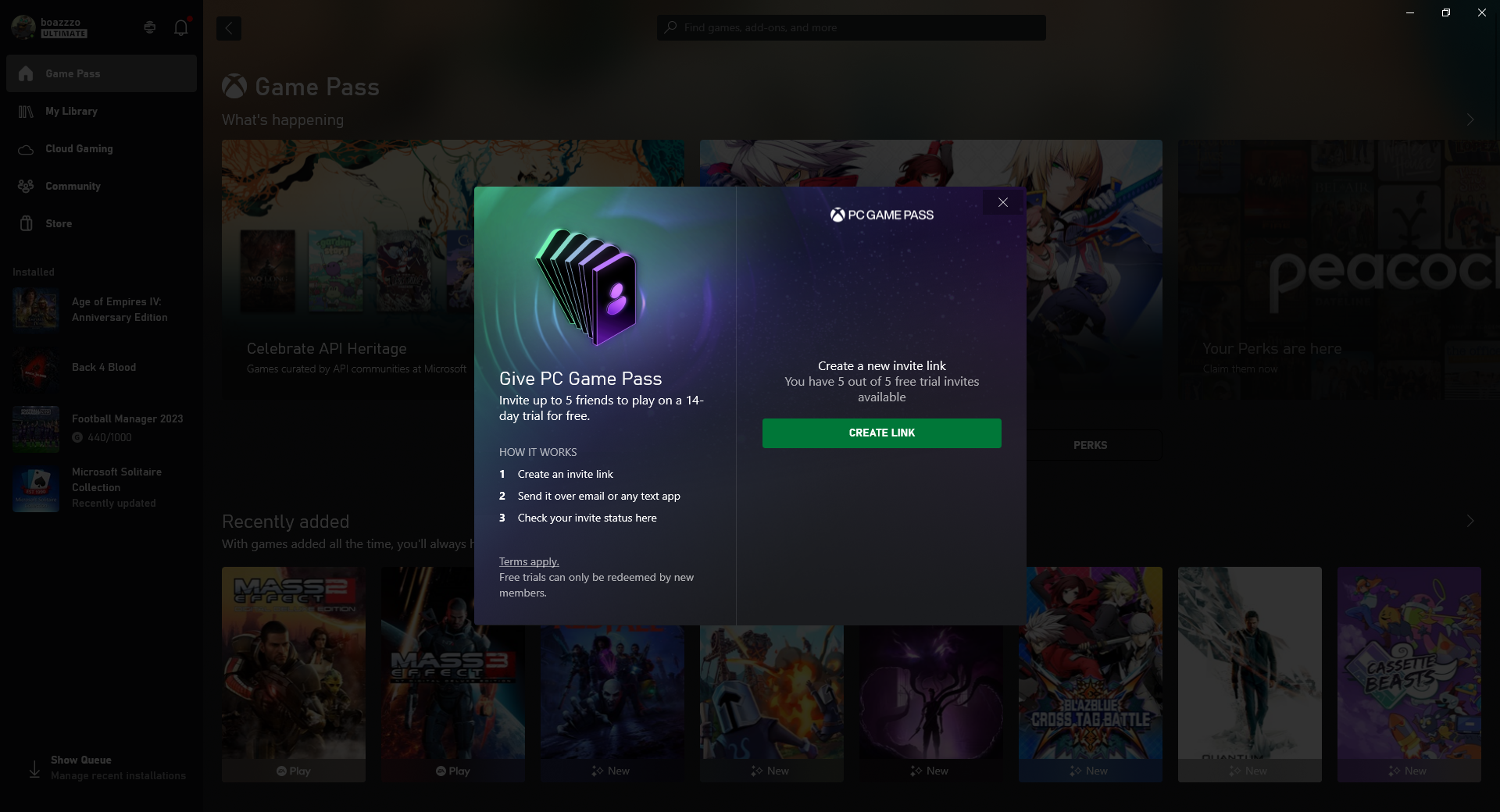A promotional pop-up for the PC Game Pass service overlays the standard Xbox Game Pass interface. The pop-up is segmented into an informational guide and an invitation tool. On the left side of the pop-up, small purple and green icons resembling phones are displayed, indicating options for user interaction. The message reads: "Give PC Game Pass: Invite up to 5 friends to play on a 14-day trial for free." It explains the process in three steps:

1. Create an invite link.
2. Send it via email or any text app.
3. Check your invite status here.

A note on terms states: "Terms apply. Free trials can only be redeemed by new members."

On the right side, users are prompted with: "Create a new invite link. You have 5 out of 5 free trial invites available." A green "Create Link" button is prominently featured.

Behind the pop-up, the Xbox Game Pass interface is partially visible. Users can see various game thumbnails including "Mass Effect" and "Mass Effect 3," "BlazBlue: Cross Tag Battle," and "Cassette Beasts." The top-right corner displays the Peacock app icon. The left sidebar features navigation options such as "Game Pass," "My Library," "Cloud Gaming," and "Community Share," along with a list of installed games.